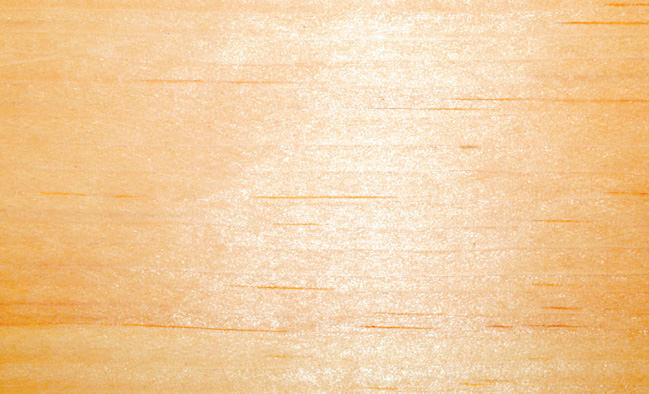This rectangular image features a smooth, light orange, almost golden yellow surface, reminiscent of plywood or a wooden table. The length of the rectangle surpasses its height. Throughout the image, thin, dark orange lines appear, running horizontally though not uniformly. Some lines are longer, while others are very short, adding a sense of texture similar to wood grain. The center of the image is visibly shinier than the edges, reflecting a light source that creates a slight white sheen, contributing to a vignette effect where the corners are less bright. Overall, the image captures the detailed texture and subtle variations in a light wood surface.